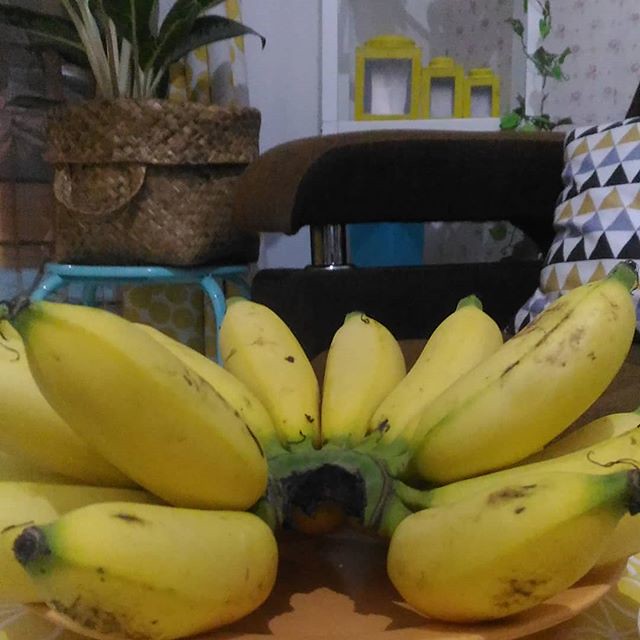In this photograph, the focal point is a bunch of bananas placed front and center, with the stem facing the viewer. These bananas are notably shorter and thicker than common varieties, giving them a rounded, almost chubby appearance. They are mostly yellow with slightly green tips near the stems and feature some black markings, indicating ripeness. To the upper left of the image, there is a teal-colored stool, on which rests a woven basket with handles. This basket contains a plant, suggesting it might be filled with soil or has a potted plant placed within it.

The background reveals more details of the setting: a blue table and a backdrop with a wallpaper pattern of white and yellow dots. There’s a decorative shelf adorned with three lantern-like objects of varying sizes—large, medium, and small—each encased in a yellow frame. Additionally, a couch with a visible armrest hosts a multicolored triangular-patterned pillow featuring shades of white, black, blue, and yellow. The overall scene is set indoors with a cozy, detailed decor that complements the central display of the bananas.